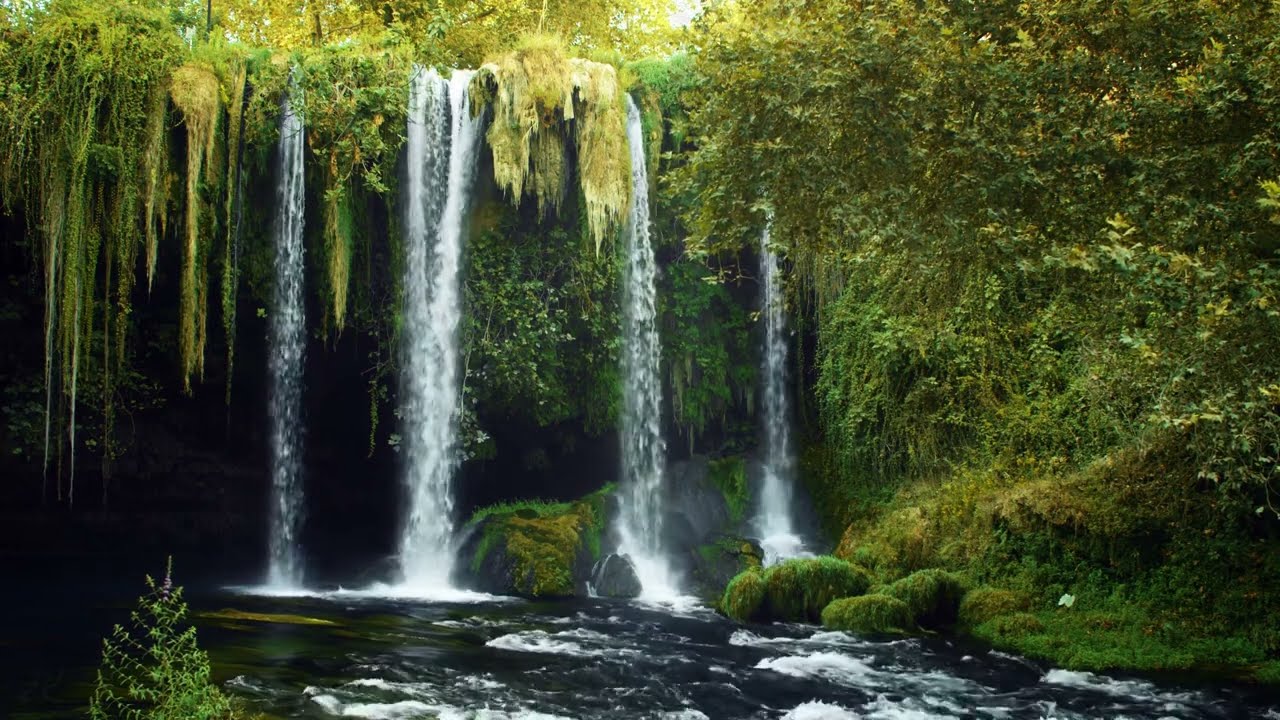This captivating daytime photograph showcases a serene natural scene abundant with vibrant green foliage. Dominated by a cascading waterfall, the image features four distinct streams of water tumbling down from a cliff draped in lush vines, ivy, and moss. Below the waterfall, a fast-moving creek or river, marked by white-capped waves and rocky edges, flows energetically. The upper portion of the shot reveals glimpses of a bluish-gray sky, illuminated by bright daylight. On the right side, there’s a large bush or tree with green and gold leaves, while the left side is adorned with Spanish moss hanging gracefully, adding to the natural beauty. A dark area behind the waterfall suggests the presence of a cave, adding an element of mystery to the scene. Overall, this image captures the tranquil yet dynamic essence of a natural waterfall amid rich greenery.